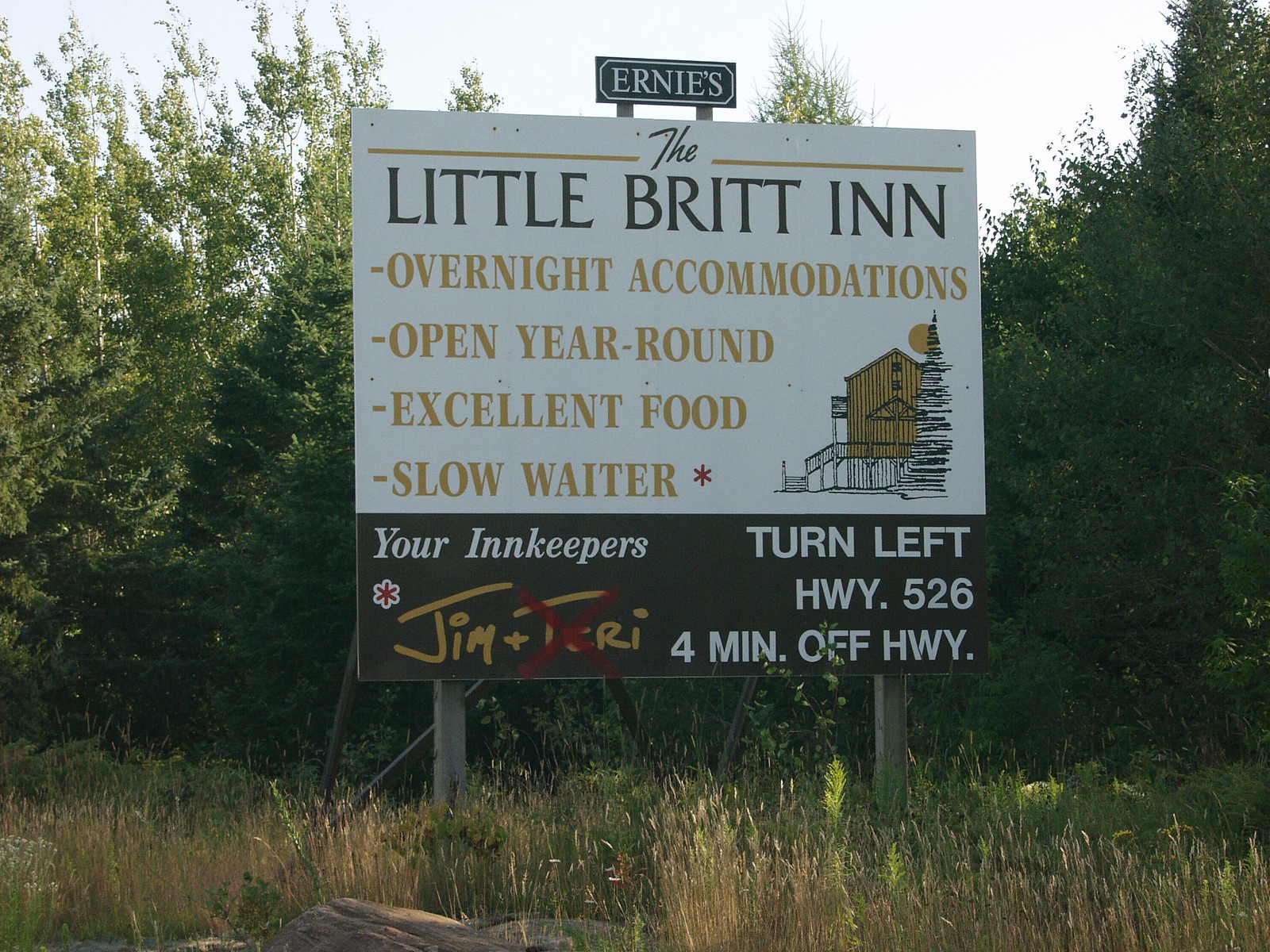This is an image of an outdoor billboard promoting Ernie's The Little Brit Inn. The top section of the billboard prominently displays the name "Ernie's" in white text on a blue mini-sign above the main portion, which reads "The Little Brit Inn" in large black font. Just below this, the sign highlights features such as "Overnight Accommodations," "Open Year-Round," "Excellent Food," and amusingly notes "Slow Waiter" in gold letters. To the bottom right of these details, there's a stylized illustration of a sunlit building and a tree, possibly representing the inn itself.

The lower section of the sign, set against a brown background, introduces "Your Innkeepers, Jim and Terry" but the name "Terry" has a red X drawn over it. Directions are helpfully provided, stating "Turn left, Highway 526, 4 Min Off Highway." The scene around the billboard includes tall beige and green grasses below, a visible rock to the lower left, and sturdy support posts visible from behind. It's set against the backdrop of a tree line under a late evening sky, suggesting the sign is likely positioned along a roadside.